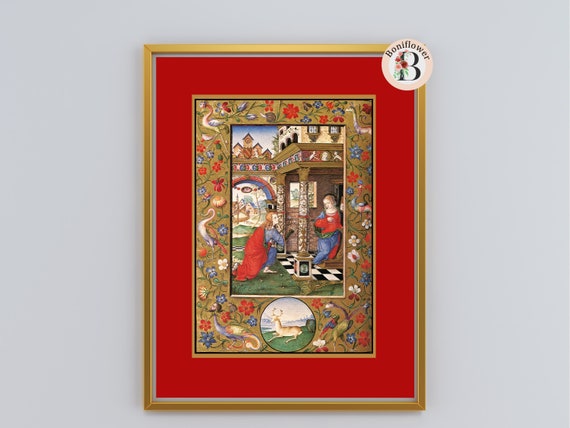The image depicts a photograph of a Renaissance-style painting encased within an elaborate multi-layered frame, hanging on a light gray wall. The outermost frame is a simple, thin, gold metallic piece. Inside, there is a large red matte board serving as a background for the inner artwork. The innermost frame is highly ornate and golden, adorned with intricate designs including flowers and various creatures—snakes, ostriches, and birds—in vivid colors such as red, blue, green, white, purple, and pink. This ornate frame also features a circular detail at the bottom, within which a deer is depicted resting on grass under a sky.

The central painting, framed within, depicts a romantic scene at the entryway of a building with pillars. A man, possibly a knight, is shown kneeling before a woman, suggesting he is trying to win her hand. Both individuals are dressed in outfits featuring blue and red hues. The setting includes a distinctive black and white checkered floor, adding to the intricate details of the artwork.